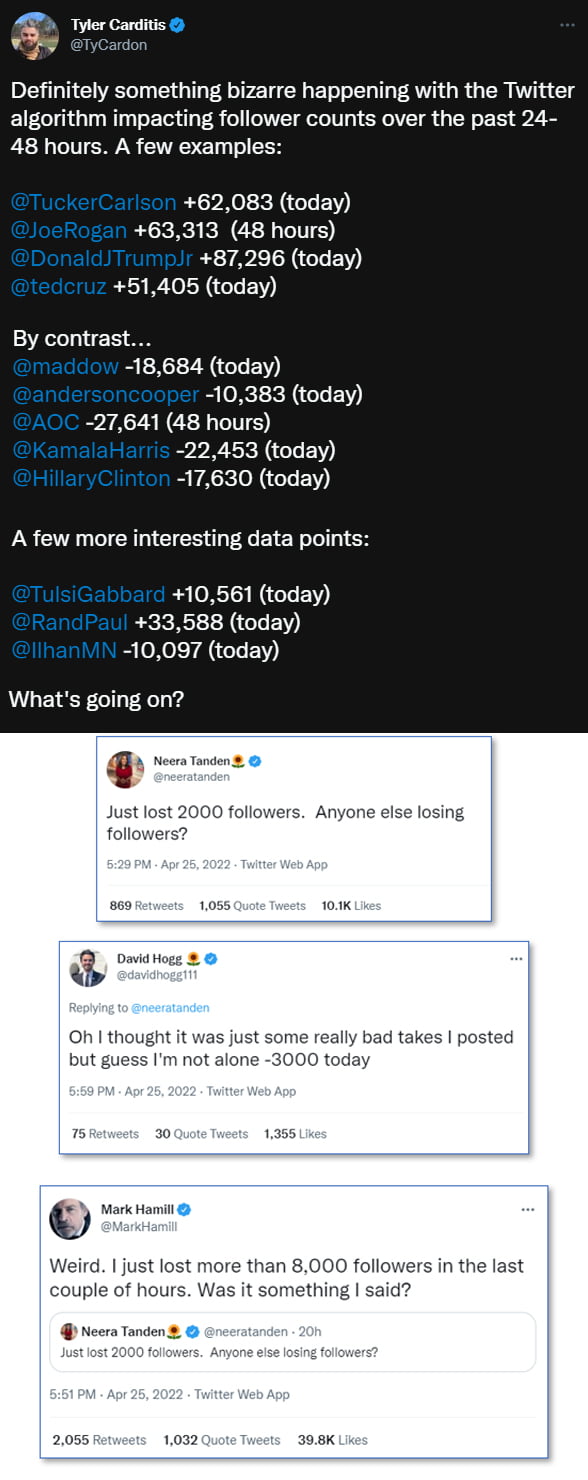**Detailed Description of the Image Captioned:**

The image appears to show a screenshot of a social media post or comment, displayed within a web interface. At the top, there's a black rectangular header, horizontally oriented, containing white text. The text reads: "Tyler Carditis." Below this heading is a summary of observed changes in Twitter follower counts, indicating unusual activity over the past 24 to 48 hours. The data points are presented as follows:

- **Positive Follower Changes:**
  - Tucker Carlson: +64,083 today
  - Joe Rogan: +63,313 48 hours ago
  - Donald Trump (@DonaldTrump): +87,296 today
  - Ted Cruz (@TedCruz): +51,405 today
  - Tulsi Gabbard (@TulsiGabbard): +10,561 today
  - Rand Paul (@RandPaul): +33,588 today

- **Negative Follower Changes:**
  - Rachel Maddow (@Maddow): -18,684 today
  - Anderson Cooper (@AndersonCooper): -10,383 today
  - Alexandria Ocasio-Cortez (@AOC): -27,641 48 hours ago
  - Kamala Harris (@KamalaHarris): -22,453 today
  - Hillary Clinton (@HillaryClinton): -17,630 today
  - Ilhan Omar (@IlhanMN): -10,997 today

The post ends with an intriguing question: "What's going on?"

This detailed breakdown helps illustrate the significant fluctuations in follower counts of various high-profile individuals, potentially indicating a disruption or anomaly within Twitter's algorithm.